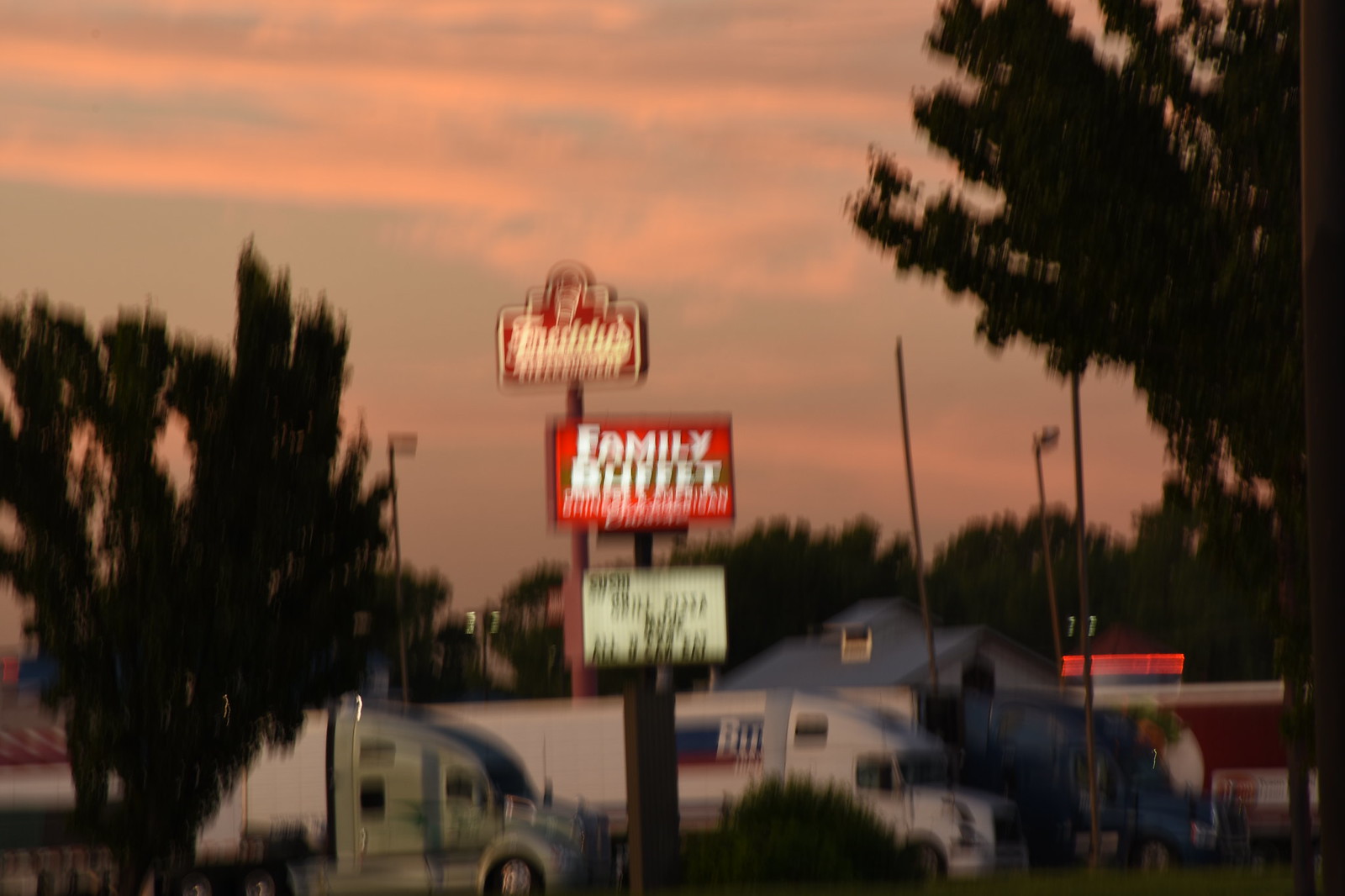In this rectangular photograph capturing either a sunset or dawn, vibrant pink and blue hues paint the sky over a busy truck stop area. Two semi-trucks, parked facing eastward in the parking lot, dominate the foreground. A slightly blurred sign in the middle ground, illuminated against the dusky sky, displays the names "Family Buffet" and "Freddy's" in prominent, lit letters, with an additional word "Sushi" below in black letters on a white background. Along the left and right sides of the image, lush green trees frame the scene, adding depth and contrast. In the lower right background, the white roof of a house peeks out from beyond the last semi-truck, providing a hint of suburban surroundings. A dark, shadowy figure, possibly a van or another semi-truck, obscures the lower right corner, adding an element of mystery to the scene.